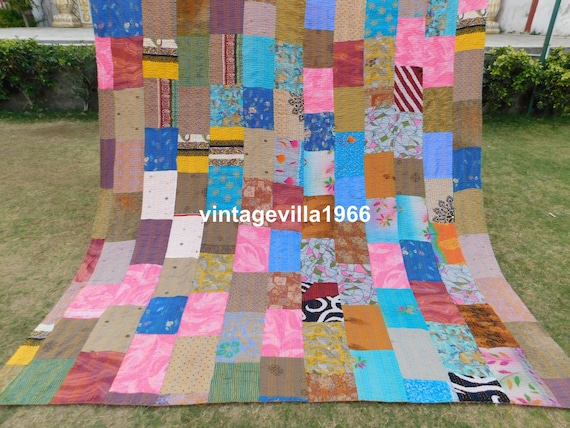This photograph showcases a handmade patchwork quilt, prominently labeled in the center with white lettering that reads "Vintage Villa, 1966." The quilt, composed of true remnants and scraps of various fabrics, is laid out on a lawn with a hedge and street visible in the background. The predominant colors are tan, pink, and aqua blue, intermixed with red, cranberry, black, and other shades like magenta, white, and brown. Each rectangle features distinct patterns, including floral designs, ocean-like motifs, wallpaper clippings, kaleidoscopic visuals, polka dots, and gradient shades, all arranged in a brick-like pattern. The quilt's diverse elements, though clashing, give it a unique character. It appears to be hung from a pole or similar structure, cascading towards the viewer on the grass, some parts of which are visibly dying with patches of green. This detailed display suggests it is a product photograph, possibly for an Etsy shop named "Vintage Villa."